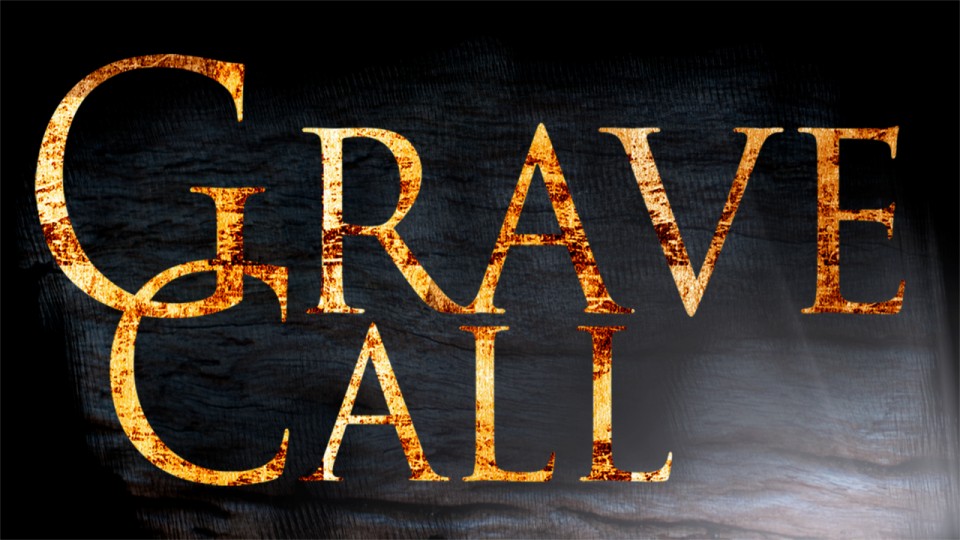In the image, the striking title "Grave Call" is written in a serif font, appearing in a rustic, goldish-yellow hue with specks of brown that make the letters look like they are burning or were once embers. Positioned prominently in the center, "Grave" is stacked above "Call," with the "C" in "Call" intricately hooking around the "G" in "Grave," creating an interconnected and eye-catching design. The background further enhances the haunting atmosphere; it is a textured, foggy gray surface that could evoke the feeling of a shadowy cave or perhaps evoke the surface of a graveyard stone. The bottom right corner of the background is illuminated, revealing more of the rock-like structure, while the top left is enveloped in darkness, adding to the eerie. The dimensions of the image are akin to a widescreen, high-definition television set, wider than it is tall, capturing the ominous essence perfectly.